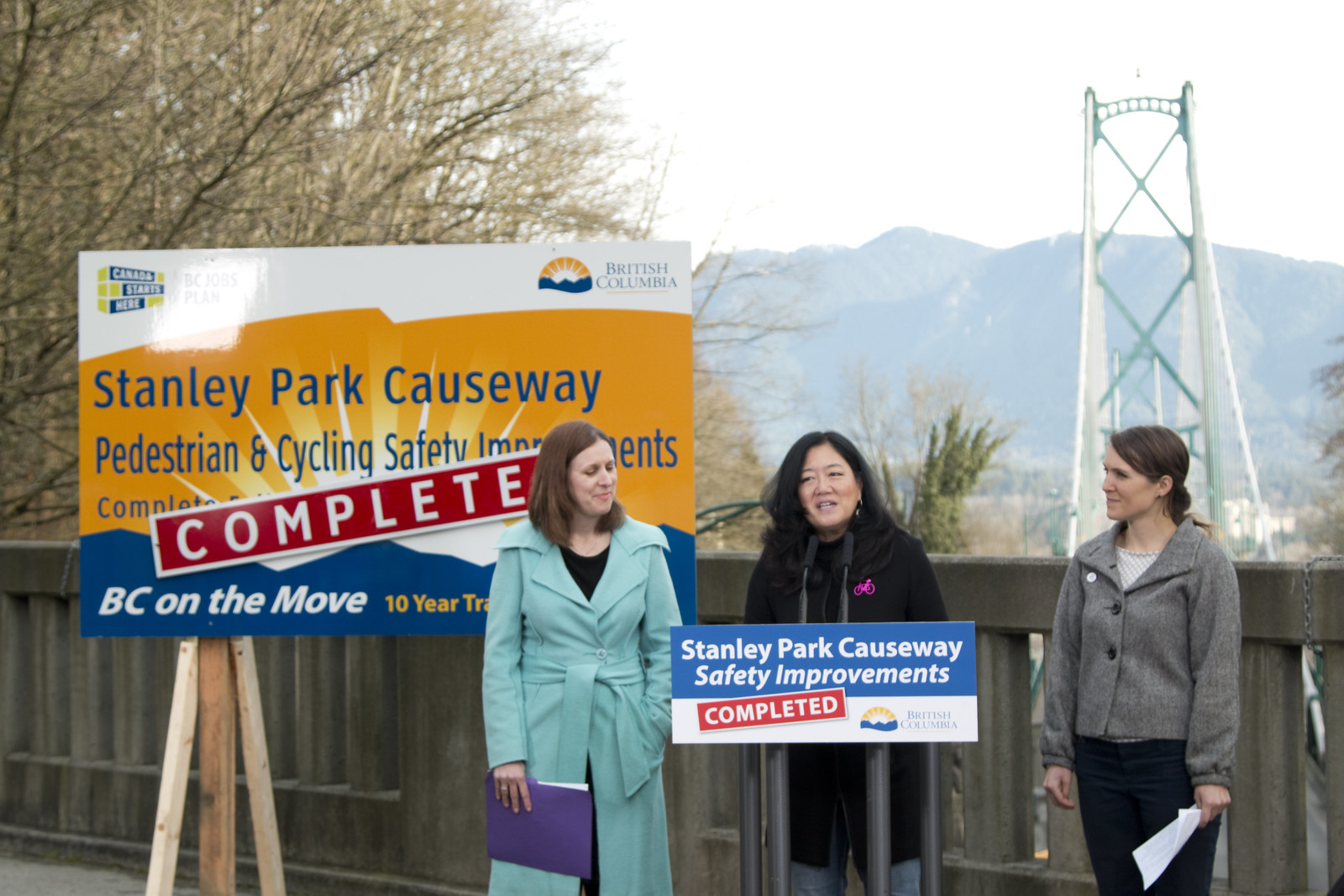This photograph captures an outdoor scene of three women standing at a podium, making an announcement about the completion of safety improvements for the Stanley Park Causeway. The women are positioned on a structure that appears to be a bridge, as behind them are the imposing towers of the bridge, with a backdrop of grayish-blue hills or mountains under a hazy spring sky. There are also some bare trees to the left, just beginning to show early spring blooms.

The woman at the center of the trio, who seems to be delivering a speech, has long black hair and is wearing a dark, likely black, overcoat. In front of her on the podium is a prominent sign reading "Stanley Park Causeway Safety Improvements," with a red rectangle at the bottom containing the word "Completed" in white letters.

To the center speaker's left stands a woman in a light greenish-turquoise overcoat, her brown hair cut to neck length, looking attentively towards the speaker. To the right is another woman with brown hair tied back, clad in a gray jacket and black pants, holding sheets of paper in her hand.

Additionally, behind the group is a large blue and white sign with the same text about the safety improvements. It also features an emblem in the corner that reads "British Columbia" and "BC on the move," along with gold lettering partly obscured by the woman on the left, indicating it is part of a 10-year initiative.